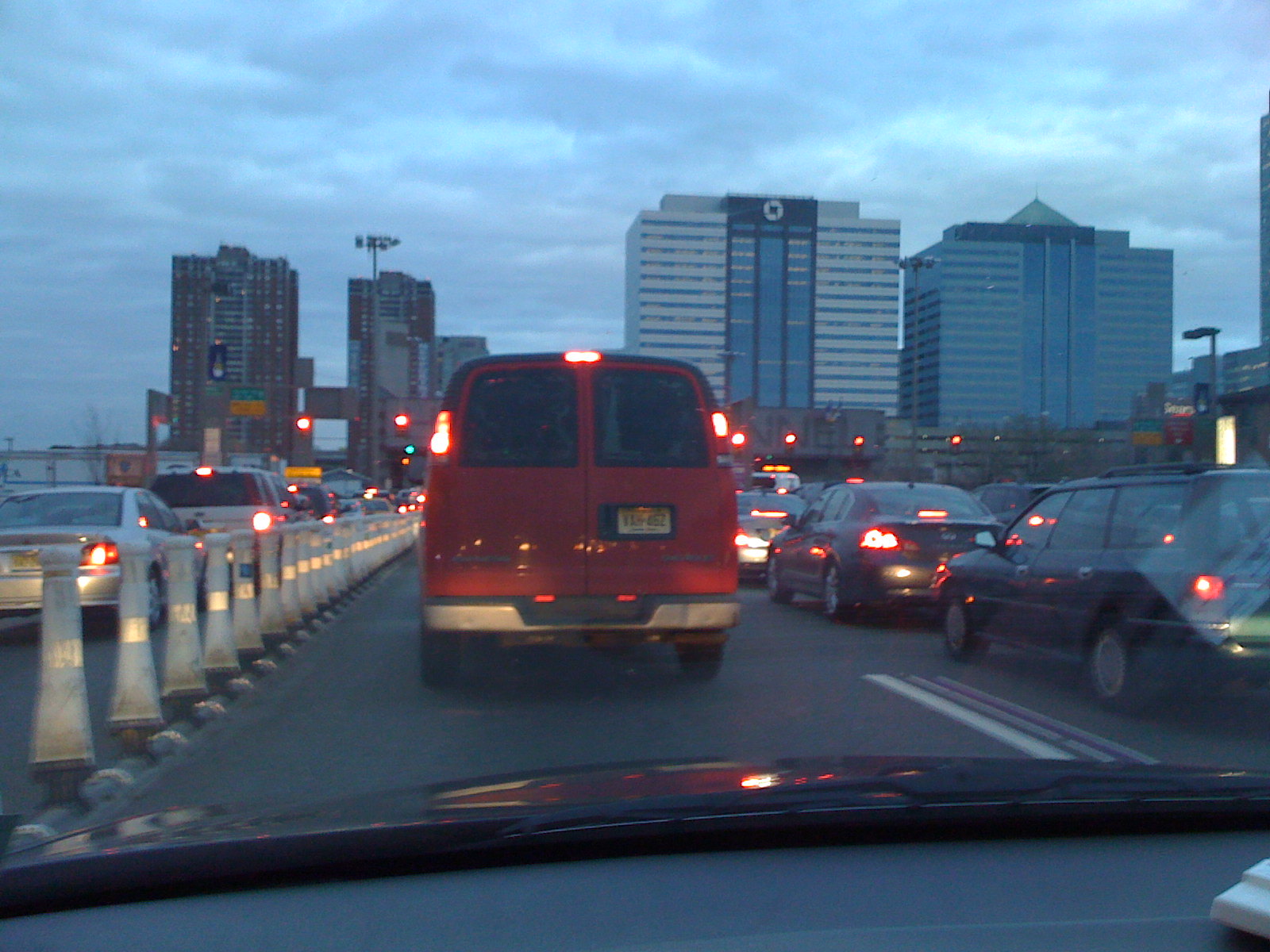A busy urban street teeming with traffic captures the essence of rush hour. Vehicles of various sizes and colors converge, including a prominent red van that stands out among the sea of cars. The atmosphere is abuzz with the hum of engines and the intermittent honking of horns, encapsulating the hustle and bustle of city life. Buildings line the street, their facades reflecting the waning daylight, while pedestrians wait patiently at the crosswalks. The scene is a quintessential snapshot of daily urban activity, where routine encounters a brief moment of stillness as the traffic lights change.